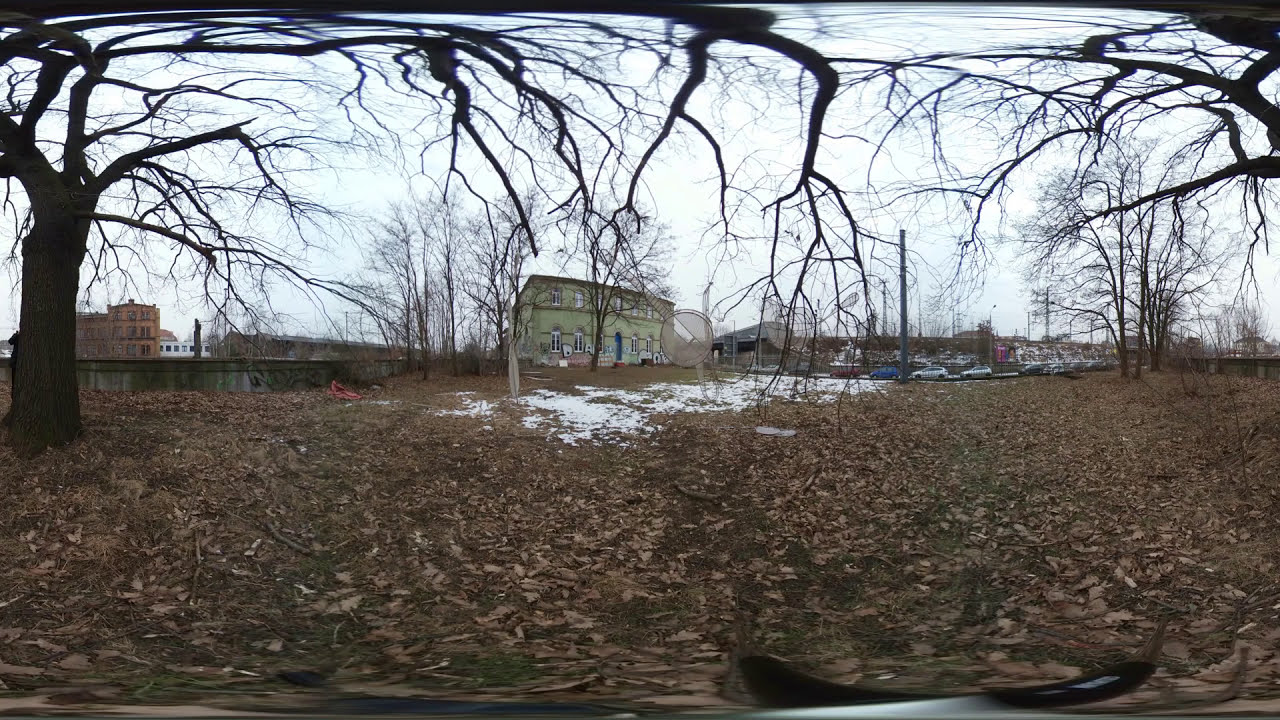The photo depicts a wintery outdoor scene characterized by a barren, brown ground scattered with dead leaves and patches of snow. The landscape is dotted with leafless trees, their bare branches stark against the overcast sky. Dominating the center of the image is a two-story building with a green exterior and numerous windows. The bottom floor features blue doors positioned slightly to the right of the center, flanked by multiple windows. To the left of the building stands a large tree whose long, branch-laden limbs stretch across the frame. Various cars, including a red one, a blue one, and several silver ones, are parked around the scene, indicating a parking area. In the background, smaller buildings can be glimpsed beyond a cement wall, adding depth to the wintry tableau.